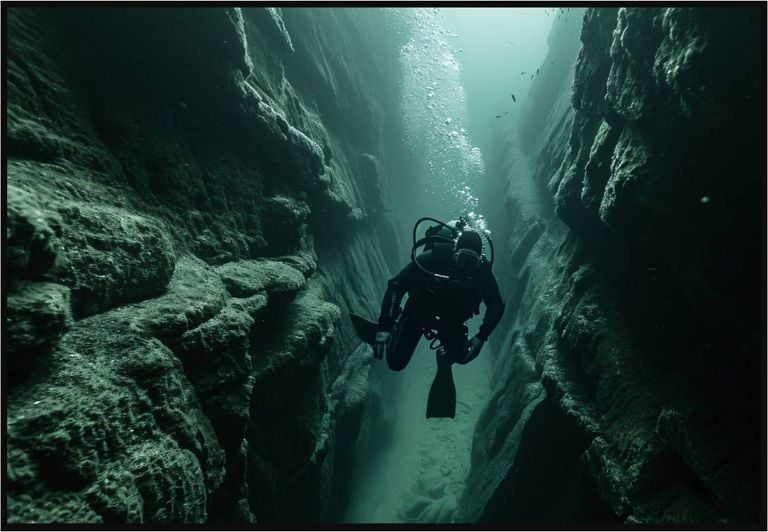This underwater photograph captures a skin diver swimming through a dimly lit, cave-like environment. The scene is predominantly dark blue and green, with gray and cloudy water adding a mystic aura. The diver, who appears to be a man based on his body size and hands, is equipped with a full set of scuba gear: a black diving suit, flippers, a full-face mask, and an oxygen tank on his back. He is swimming toward the camera, situated between two jagged, curvy stone walls that resemble rocky cliffs, wider at the top and narrowing near his position. Bubbles emanate from his breathing apparatus, trailing upwards as they ascend to the surface. The ground beneath him is sandy and light green in color. The cave's ambiance shifts from dark greens and blues to a brighter upper section, implying that the water's surface is not far above. The photograph vividly portrays the diver's journey through this mysterious underwater corridor.